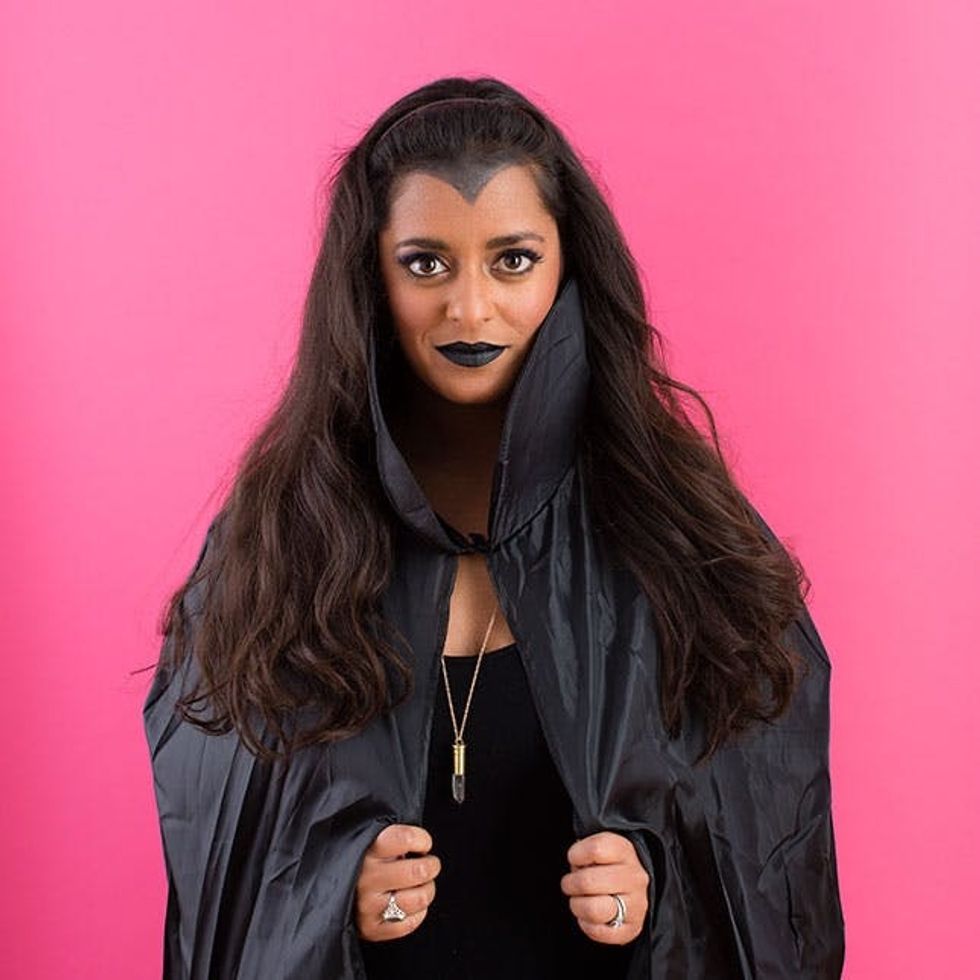In the photo, a young lady, dressed in what appears to be a gothic or vampire-inspired costume, stands confidently against a vibrant pink background. She is adorned in a black gown with a matching high-collared cape and black lipstick. Her makeup includes a distinct widow's peak design, adding to her vampiric appearance. She possesses striking brown eyes, accentuated by expertly done eyelashes, and long, flowing black hair.

On each ring finger, she wears a ring, and around her neck dangles a necklace with a charming crystal pendant. Her complexion is tan, which contrasts beautifully with her dark attire. The vivid colors of the scene include bright pink, tan, silver, gold, black, and white, creating a striking visual contrast. The woman gazes directly at the camera, holding the edges of her cape with both hands, emphasizing her dramatic and alluring pose, suitable for an alternative modeling setting or a Halloween-themed photo shoot.